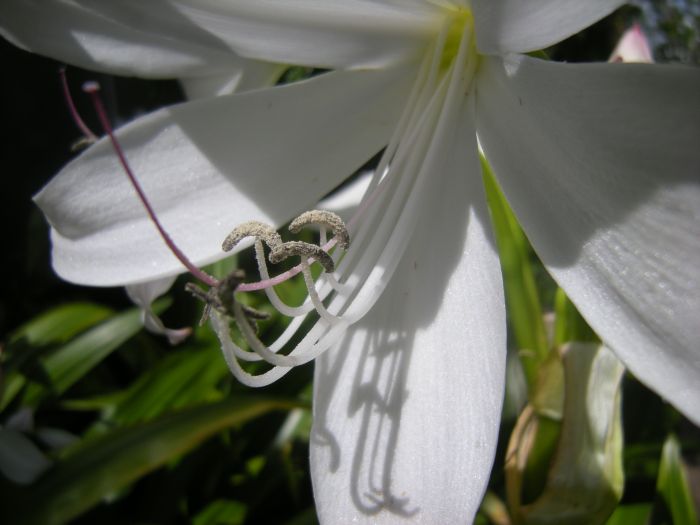This is a detailed close-up photo of a white lily flower. The image prominently features the central part of the flower, showcasing the yellow middle and at least six visible petals, some partially extending beyond the frame. Emerging from the center are multiple stamens and a purplish pistil, with noticeable pollen adorning the tips of the stamens. The lily's petals display a wet-looking, though not velvety white surface, with subtle hints of yellow towards the center. The flower is bathed in sunlight, casting deep shadows that suggest the photo was taken around midday. In the background, there's a mix of blurry hints of other flowers, dark green shiny foliage, and a blend of green, dark shades, and a touch of blue, possibly representing the sky. The overall scene implies that the flower is still part of a living plant, as opposed to being cut and placed in a vase.